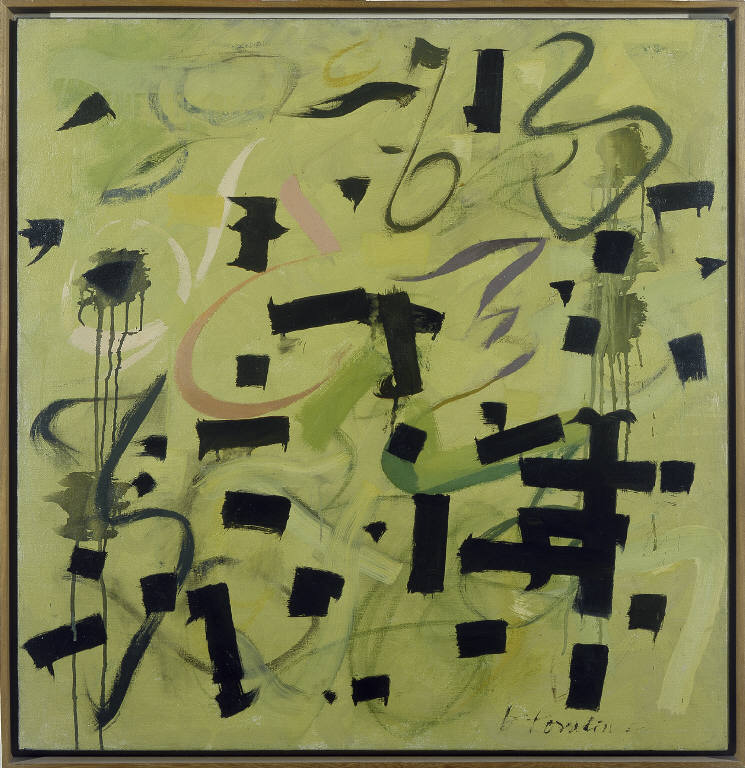This abstract painting, nearly square in shape, features a mottled background with shades of yellowish-green and olive green. The canvas is set within a thin brown wooden border, adding to its framed appearance. The background is adorned with intricate, calligraphic squiggles and splotches of various colors including white, pink, light red, bluish, and purplish hues. These squiggles are thin, calligraphy-like lines that vary in thickness. In contrast, there are bold, thick black streaks that dominate much of the canvas, accompanied by some gray ones, creating a striking visual contrast. Most of these black strokes are straight lines with some interconnected patterns, particularly concentrated in the bottom right corner. Across the canvas, there are also lighter streaks of purple, blue, and additional white elements that add nuance to the overall composition. In the center of the painting, patches of pink, peach, and white contribute to the abstract aesthetic. Notably, the upper part of the painting features strokes resembling the number '63'. The bottom right corner is signed in black, though the signature is ambiguous, possibly reading something like "Torah Tim" or "V-T-O-R-O-T-I-N". The entire arrangement presents a dynamic, almost chaotic visual experience, reminiscent of a jumbled collage of various tones and textures.